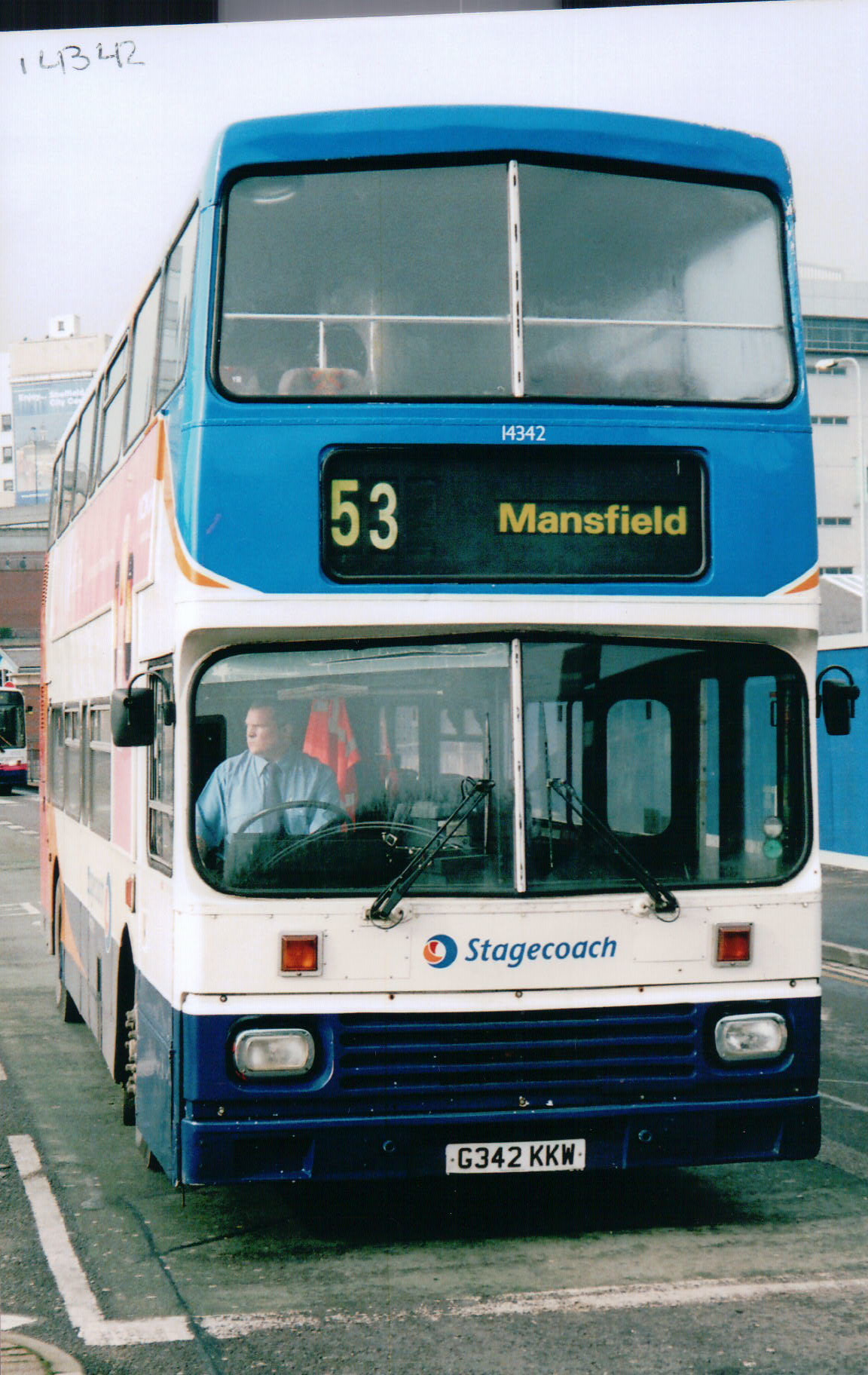This detailed image shows the front view of a bright turquoise blue, double-decker Stagecoach bus, numbered 53 and heading to Mansfield, according to the black label with yellow lettering at the top of the bus. The bus is parked on a pavement area, with a hint of another bus visible behind it and some buildings in the background. The driver, seated on the left side, is seen wearing a light blue, long-sleeve shirt with a dark tie. In front of him, the white portion below the windshield is emblazoned with the "Stagecoach" logo. Flanking this are two square, red lights. Below this section, the grille is navy blue with two white headlights and a white license plate reading G342 KKW. The bus has a striking combination of blue and white elements, with the driver's position and visible details adding to the overall composition.